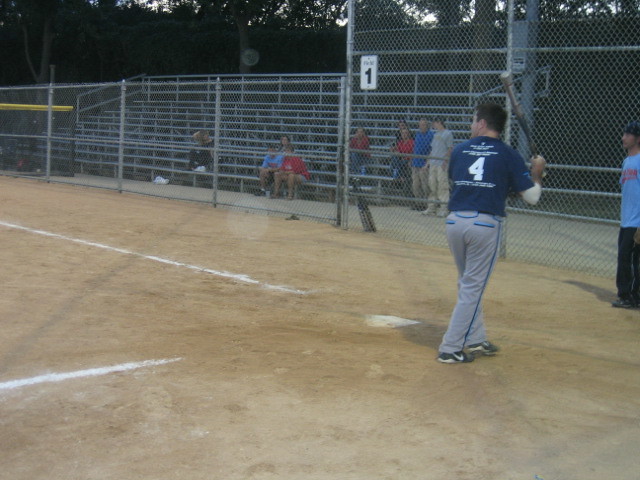This image captures a man at bat during a baseball game, poised and ready to swing. He is wearing a navy blue short-sleeved shirt, with the number 4 prominently displayed in white on the back. Bold white lettering is also present above and below the number, though it is unclear. He is dressed in gray baseball pants that feature light and dark blue stripes down the sides and around the pockets, paired with black cleats. The man's right arm is bent slightly behind him, gripping the bat.

In the background, a chain-link fence extends from the middle of the left side and continues off the top of the screen. There is a metal sign with the number 1 on the left part of the fence. Behind the fence, silver bleachers are occupied by about ten spectators, seemingly family members, some standing and others seated. Farther back, a tree line is visible, with patches of light filtering through. The batting area below consists of dirt, with diagonal white lines representing the batter's box, converging towards a white home plate. On the far right edge of the image, partially visible, stands another man or boy in a light blue shirt and black pants.